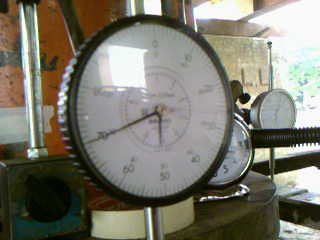The image depicts a vintage weighing scale situated in an outdoor area, evidenced by the background on the right, which reveals an open space adorned with trees and bathed in sunlight. Front and center stands the scale, which prominently features a large dial displaying a weight of 70 units (the specific measurement is unclear due to a lack of detail). The main dial, characterized by its large white face with black numbers, is partially blurry, obscuring the model and brand name. A smaller second dial is situated within the larger dial, while an inner black circle contains indecipherable markings. The outermost edge of the scale's face is framed by a textured black rim that resembles the crimped edge of a bottle cap, all mounted on a silver pole.

Adjacent to the scale, on the left, is an old rusted metal box with remnants of blue paint and a circular feature protruding from its center, potentially a piece of wood, suggesting it might be a heater. A silver pipe extends from the top of this box. The backdrop consists of an orange wall marred with black and white stains, indicating significant wear and tear.

Directly behind the main scale dial, a large round object that appears to be a roll of masking tape is visible, alongside a silver tube containing an unknown substance. These items rest on a cement stand. Another similar dial is partially obscured behind the main scale, and further to the right, yet another dial is seen, affixed to a silver pole extending both above and below it. A large black bar intersecting the scene in the foreground suggests the setting is a mechanical workshop, reinforcing the industrial ambiance of the image.